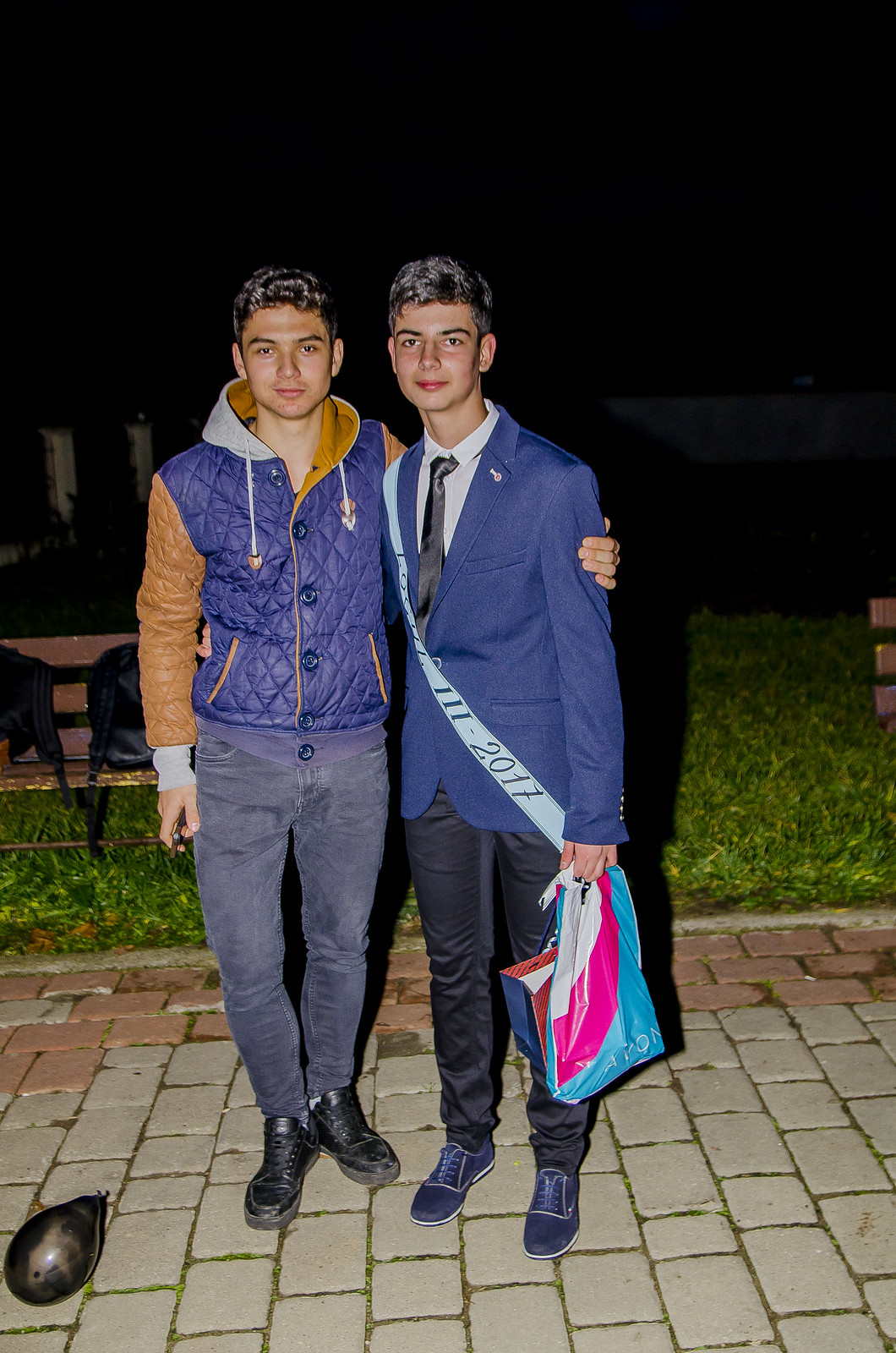This photograph depicts two young men standing close together and posing for the camera with their arms around each other. Both appear to be in their late teens or early 20s and are of Caucasian ethnicity. They are outdoors at night, as evidenced by the dark background and the use of a camera flash. They stand on a brick-paved walkway with patches of green grass visible behind them, along with a small park bench.

The man on the left is wearing a distinctive purple and orange jacket with a hood, paired with a purple shirt underneath, blue jeans, and black shoes. He has short brown hair and is clean-shaven. His left arm is draped over the shoulder of his friend on the right, while his right arm hangs relaxed at his side. Additionally, there is a strap crossing from his right shoulder to his left hip, and a pin is attached to his jacket.

The man on the right is dressed more formally in a blue suit jacket, a white button-down shirt, and a dark tie. His ensemble is completed with black trousers and dark shoes. He, too, has short brown hair and is clean-shaven. A distinctive sash across his chest reads "2017," and there is a pin on his jacket. He is holding a multicolored bag, which is pink, light blue, and white, in his left hand. The relaxed posture of his left arm suggests a comfortable and friendly pose with his companion.